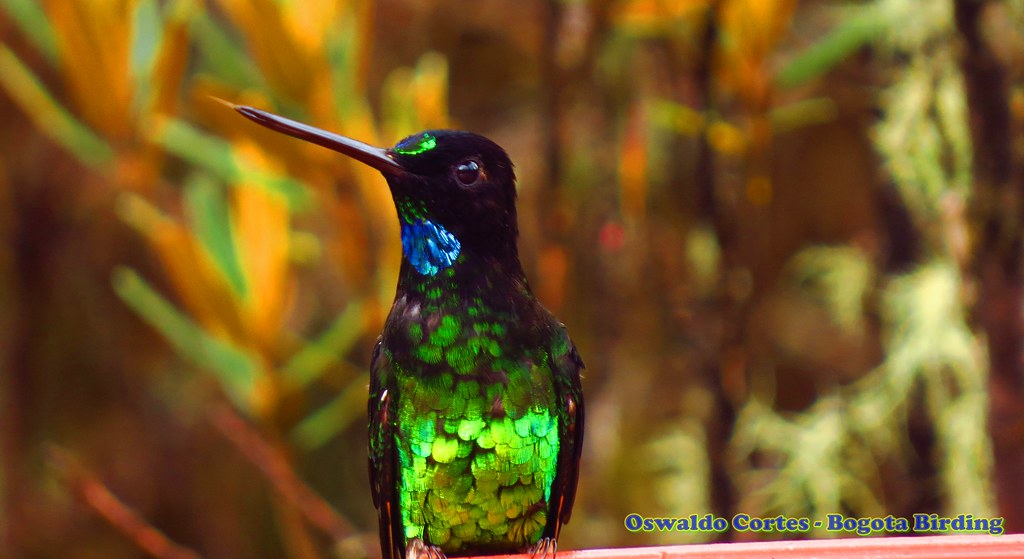This detailed and vibrant photorealistic image, possibly enhanced with filters for increased saturation, showcases a striking bird perched at the center. Although likened to a hummingbird due to its slim, dark, and elongated beak, the bird features unique neon accents that set it apart. Predominantly black, its plumage is adorned with a shimmering array of colors: a bright green forehead spot, a vivid blue patch under its chin, and a chest covered in bright green feathers speckled with brown and black. Its wings, though not fully visible, appear to continue the pattern of brown and green speckling.

The bird is perched confidently on a pink surface, perhaps a board or branch, with notable pink feet adding to its colorful appearance. The long beak, characteristic of hovering birds, extends from its face, enhancing its exotic look.

Surrounding this avian wonder is an artfully blurred background, creating a bokeh effect that suggests lush foliage in vibrant hues of green, orange, and red. Off-center, slightly to the right, a discreet yet clear credit states: "Oswaldo Cortes - Bogota Birding." This text implies that Oswaldo Cortez, perhaps a noted bird photographer, is the artist behind this remarkable capture.